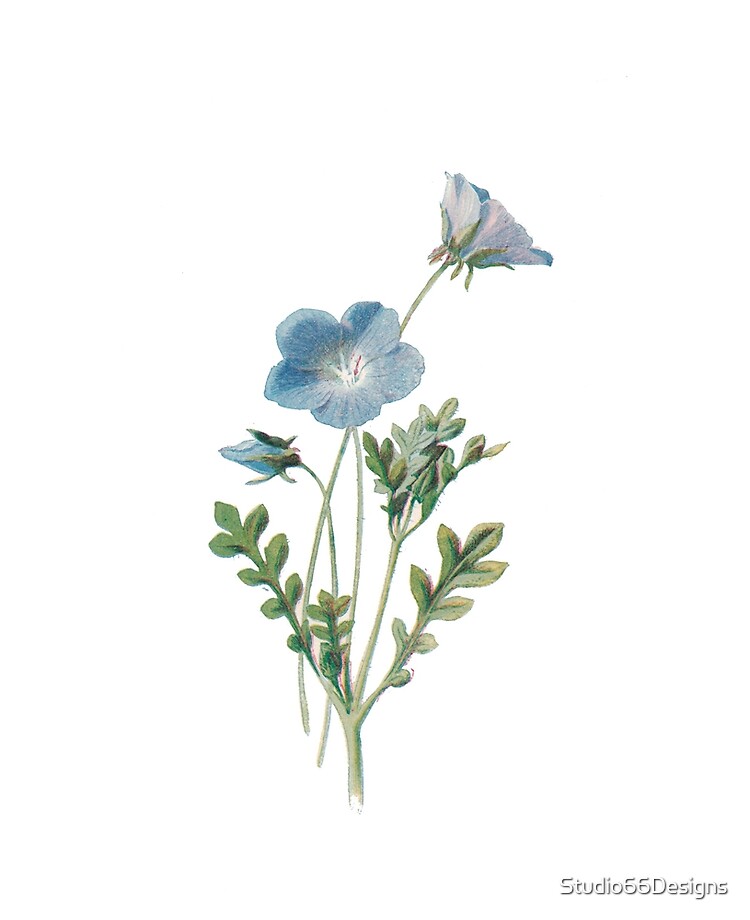This illustration, set against a clean white backdrop, showcases a simple yet elegant watercolor-like depiction of a flower. The artwork features three slender green stems and a sprig with lush green leaves. The flower's main elements are a closed bud, a fully bloomed middle flower, and an open flower shown in profile at the top. The flowers exhibit a delicate blue hue, resembling a peony, with the open blooms displaying five distinct petals. The closed bud curves downward to the left, while the top flower curves gracefully up and to the right. Marked with a “Studio 55 Designs” watermark in the bottom right corner, the image exudes a fresh, moist, and vibrant quality, capturing the beauty and simplicity of nature without any distractions.